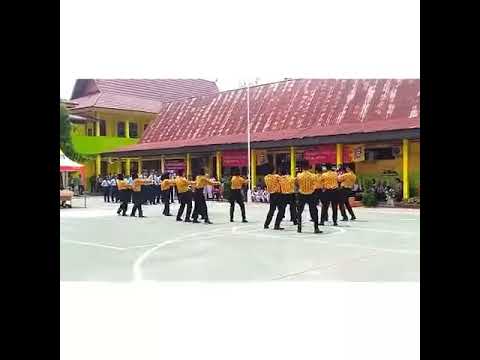The image depicts a lively outdoor event in an unspecified Asian country. In the forefront, numerous people are dancing energetically on a paved area that appears to resemble a basketball court, as indicated by visible court markings. The performers, both male and female, are dressed in coordinated yellow shirts with black pants. Behind them is a large, prominent building featuring a red, sloped roof adorned with smeared red and white vertical stripes, and supported by bright yellow pillars. The building's walls are mostly yellow with hints of green near the bottom and are decorated with red banners.

The photograph, though somewhat grainy and of older quality, captures the vibrant atmosphere as a canopy in red and white stripes shelters part of the audience. On the left side of the image, another group of individuals dressed in white shirts and blue pants stands attentively, possibly spectators or another performing group. The background reveals additional structures, including another building with yellow pillars and a similar red roof. The sky above is a flat, white expanse, indicating daytime. The detailed and structured scene highlights an event filled with coordinated groups, presumed performances, and engaged spectators, bringing a vivid sense of cultural festivity.